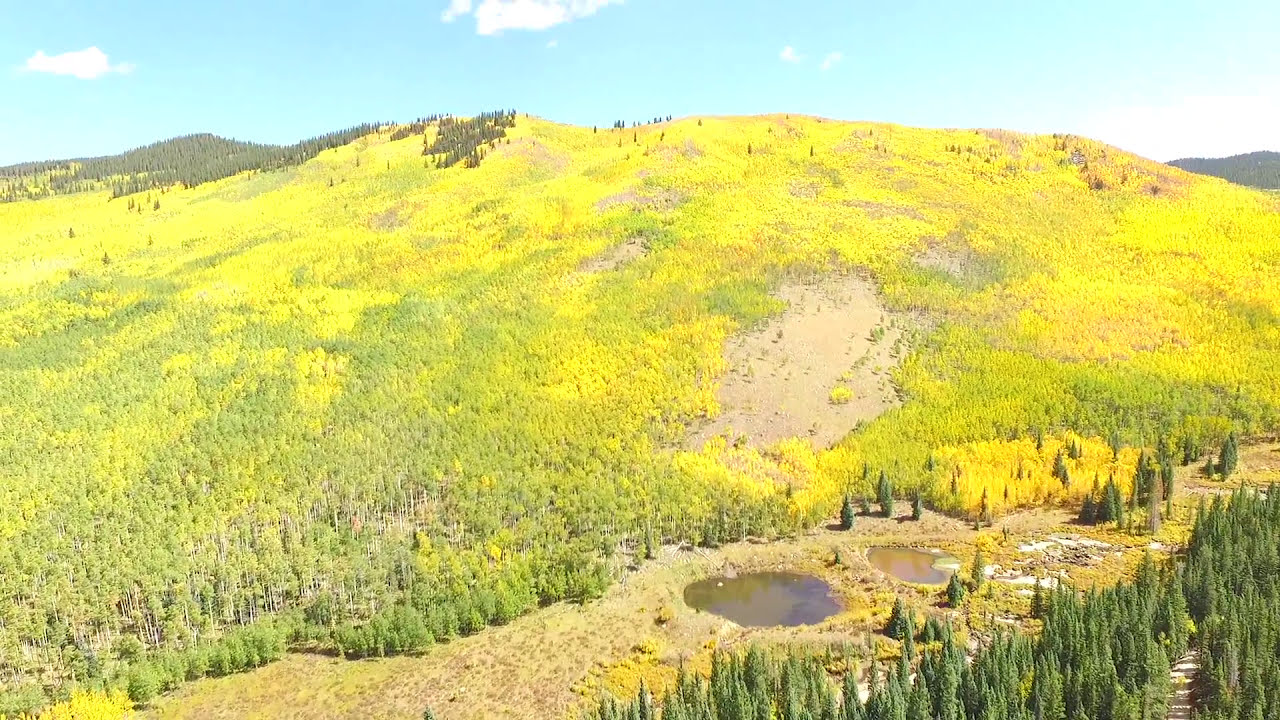The image captures a stunning, potentially Irish, outdoor scene featuring a rolling hillside. Evergreen and pine trees dominate the landscape, transitioning into deciduous trees whose leaves are a vibrant yellow, suggesting the onset of autumn. Part of the hillside is notably bare, as if a landslide has stripped away the trees, creating an odd, tree-less patch. The sky above is a clear, pale blue adorned with a few small, scattered clouds. The bottom right corner showcases dense, green pine trees, leading into a unique section with two adjacent, man-made ponds, separated by a narrow strip of earth. A noticeable dirt path, possibly an old riverbed, runs across the hillside, its brown surface dotted with a few remaining puddles, indicating recent water flow or spring snowmelt. The incline of the hill and the varying tree colors create a captivating, somewhat surreal scene that could be mistaken for an over-sharpened or manipulated image, though it maintains a realistic charm.